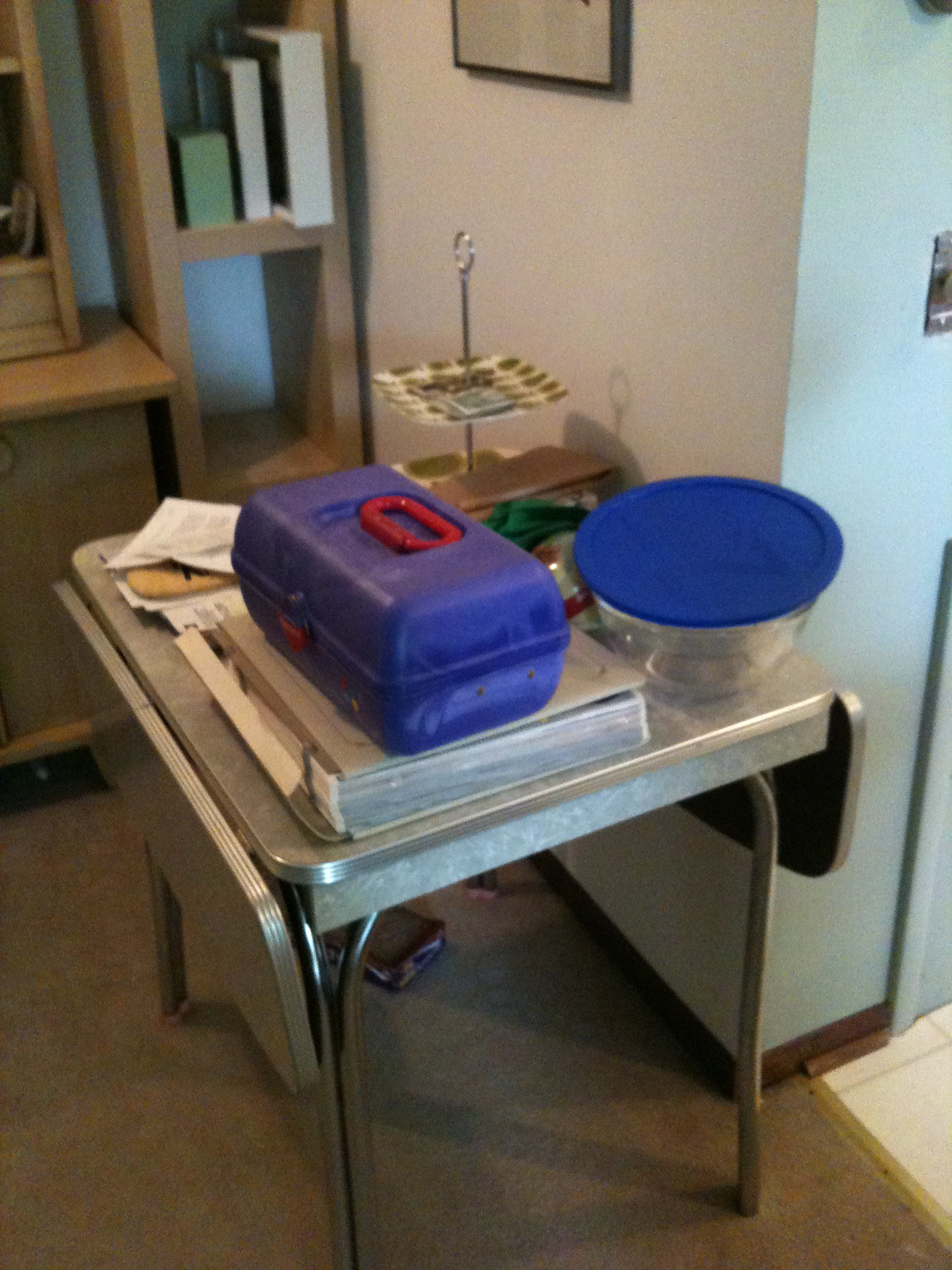The photograph captures a vintage kitchen table, reminiscent of styles from the 1950s or 60s. The table features a durable, easily wipeable plastic surface, and has two folding sides that, when down, give it a rectangular shape but can be lifted to create a square form, perfect for space-saving. The table is situated in a carpeted area, adjacent to a kitchen identifiable by its tile flooring. Behind the table stands a wooden cabinet. 

On the table, a variety of items are neatly arranged: a clear glass bowl with a medium blue lid, a thick photo album with a white cover, and a small painter’s box in medium blue with a red handle. Additionally, there is some scattered paperwork in the upper left corner. A tiered snack holder with two shelves, a silver pole, and a ring at the top completes the eclectic assortment of items on the table.